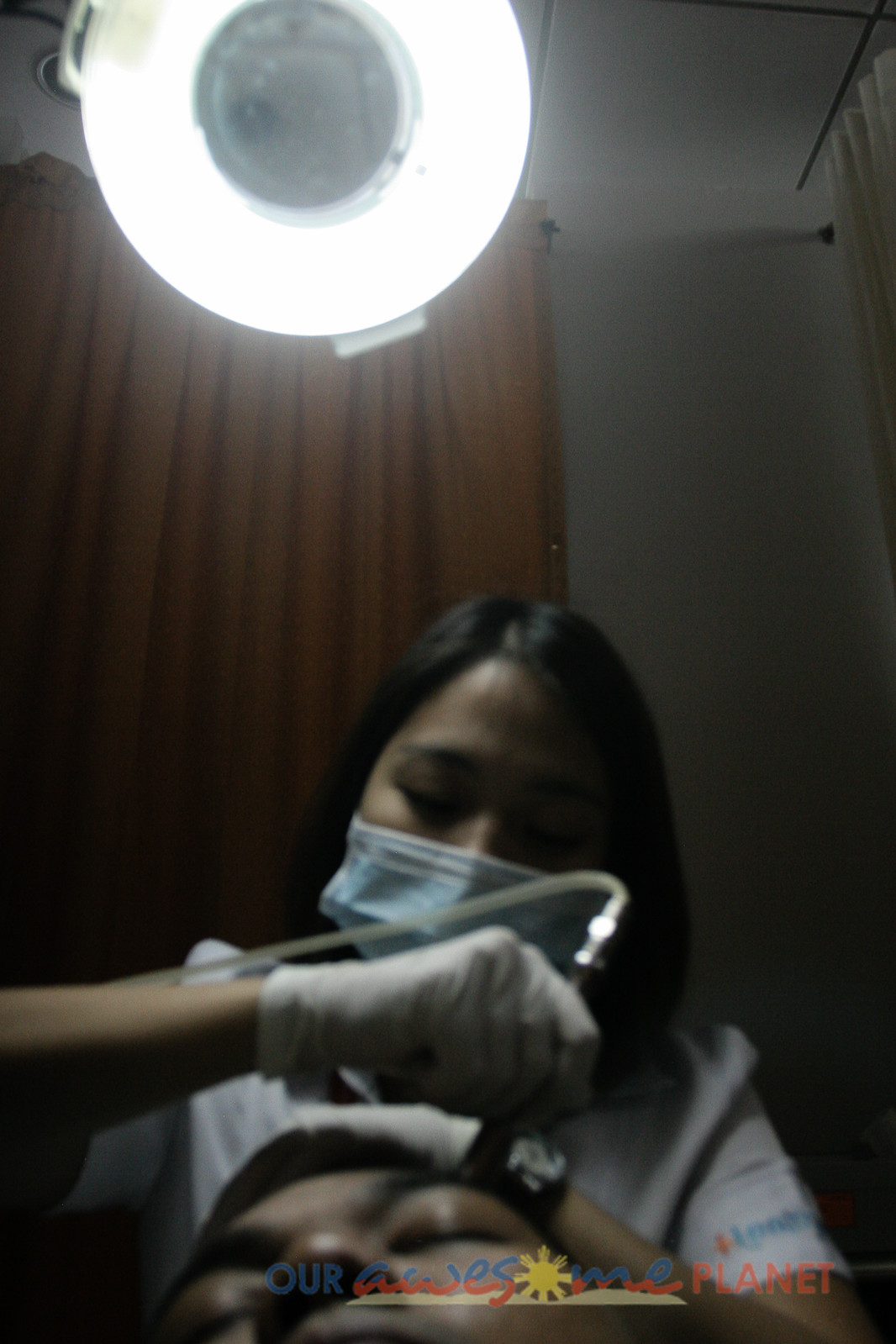In the dimly lit, vertically-oriented image, a medical procedure is taking place. The room is mostly dark save for a single, circular ring light at the top, which casts a focused glow onto the scene below. Behind the light, a pair of closed orange or red curtains contrasts against the otherwise white walls, adding a touch of color to the setting. 

At the bottom of the image, a man with closed eyes and brown skin lies seemingly unconscious, his head being the focal point of the procedure. His black hair frames his face, which is partially visible from the mouth upwards. Hovering over him is a woman who appears to be either a nurse or doctor. She has brown skin and straight black hair, partially obscured by a light blue surgical mask covering her nose and mouth. 

Dressed in white medical clothing and sporting white latex gloves, she delicately holds a silver medical instrument in her hand. This device features a transparent tube extending from it, although the exact function and endpoint are not visible. With one hand, she steadies the man's head, while the other operates the medical device, working on what appears to be the top back of his head. 

At the very bottom of the image, the text "Our Awesome Planet" is visible in blue and red letters, with the 'O' in "awesome" shaped like a yellow sun, giving the photograph an additional layer of context or branding.